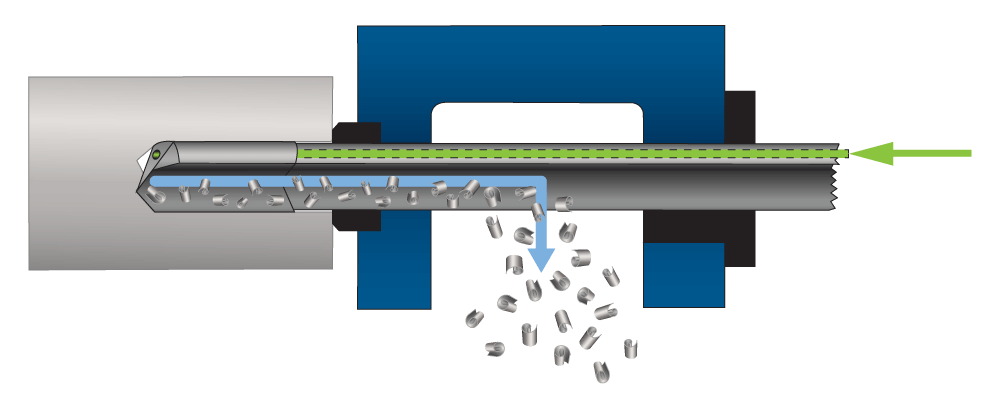This image is a detailed infographic illustration, possibly a computer animation, demonstrating the functioning of a machine or tool. The infographic features a color palette of gray, blue, green, black, and white. 

On the left-hand side of the image, there is a large gray (or silver-colored) rectangle. In the center, an arched blue framework sits with black accents on either side. The primary focus is an oblong, silo-like tool laid on its side, spanning the length of the image. This tool is gray, with significant components and highlights in blue and green. 

At the right-hand side, a green arrow directs into the tool through a metallic-colored tube. The arrow follows through the structure, guiding the eye leftward. Along this path, a green rectangle with a dotted outline possibly indicates an object or material entering the tube. 

The green arrow transitions to a light blue one at the center and points downward, indicating movement through the device. As it moves downwards, it signifies the falling of small silver or gray bits, which are finally expelled from the bottom of this conveyor-like tool. This breakdown process is underscored by the depiction of these small pieces being dropped out at the end. The background includes a mix of blue and black rectangles and supports the overall mechanical theme of the graphic.